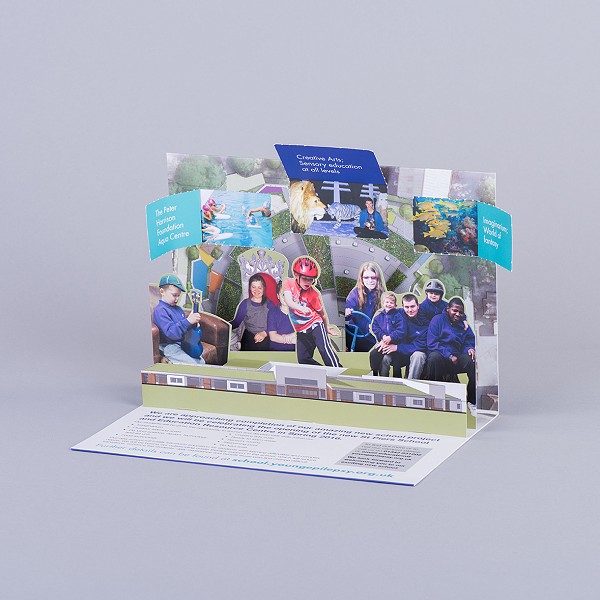This is an intricate and vividly detailed pop-up card or promotional flyer likely for a school project, featuring various hinged elements and tear-up windows that reveal additional images and text. When opened, the card displays multiple photographs depicting a range of activities and people. Central to the scene are children engaging in different activities: a young child playing a small blue ukulele while sitting in a brown leather chair, possibly wearing a hat and blue shirt with jeans; another child wearing a red helmet, involved in what seems to be a sporting activity, potentially skateboarding; and two young girls adorning a throne-like chair. On the right side of the pop-up, an adult man stands with three younger boys. Additional features include a woman steering a blue steering wheel.

The base of the card is lined with text, although much of it is difficult to decipher. Prominent readable phrases include "Father Harrison Foundation Aqua Center," "Creative Arts Seminary Education at All Levels," and "Imagination World of Fantasy." Each phrase is associated with a folded flap, revealing further illustrative details beneath: people swimming in a pool for the Aqua Center, a person flanked by a lion and a white tiger for the Creative Arts section, and various fish swimming for the Imagination World of Fantasy. Overall, the card is an engaging, multi-layered depiction of educational and recreational activities, suggesting it is a creatively designed promotional piece.